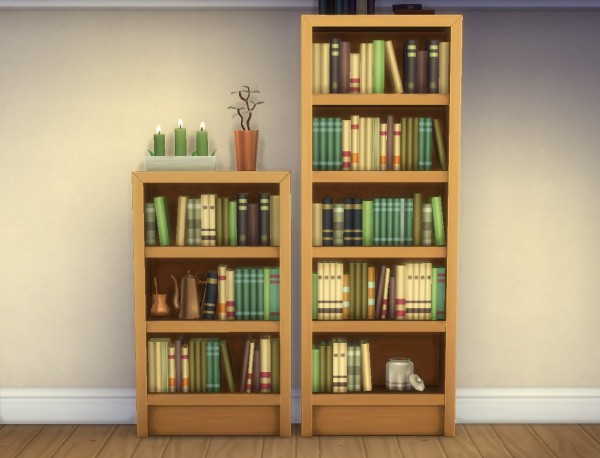The indoor setting of this flat features two distinct bookshelves against a tan wall with a white baseboard, resting on wooden floorboards. On the left, a shorter bookshelf with three layers holds a multitude of books. Atop this left shelf, a white tray bears three lit green candles of varying heights—the middle candle being the tallest, the left the shortest, and the right the second tallest. Adjacent to the candles sits a bronze pot containing a bonsai-like plant with a few green leaves. The right bookshelf stands taller with five layers, nearly reaching the ceiling, and is similarly filled with numerous books. The top of this taller shelf displays an assortment of items, including a bowl and other indistinguishable objects. The overall scene, likely a computer-generated image, captures a cozy and detailed interior design.